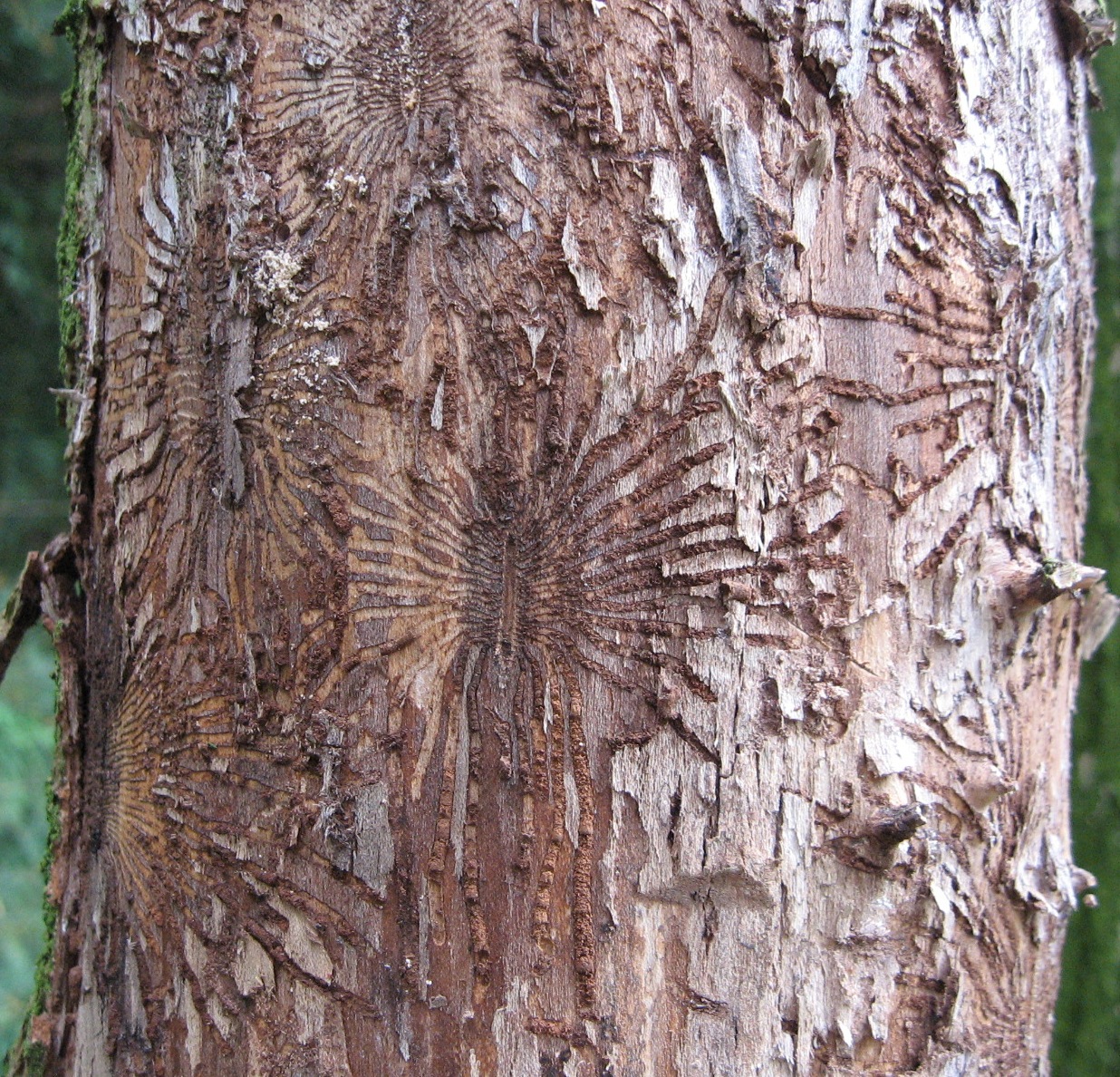This close-up photograph captures the middle section of a large tree trunk, prominently displaying its textured bark. The bark features intricate carvings or markings, which consistently resemble fossilized insects with distinct bodies and radiating legs. While the tree trunk is mostly brown with various shades, some sections of the bark appear to be peeling, and there is a noticeable patch of green moss on the left side. The background reveals a hint of greenery, placing the tree in an outdoor setting. The precise alignment and design-like appearance of the carvings make it difficult to determine if they are naturally formed or man-made. The right edge of the photo shows the tree’s original bark intact, adding to the complexity and beauty of the image.